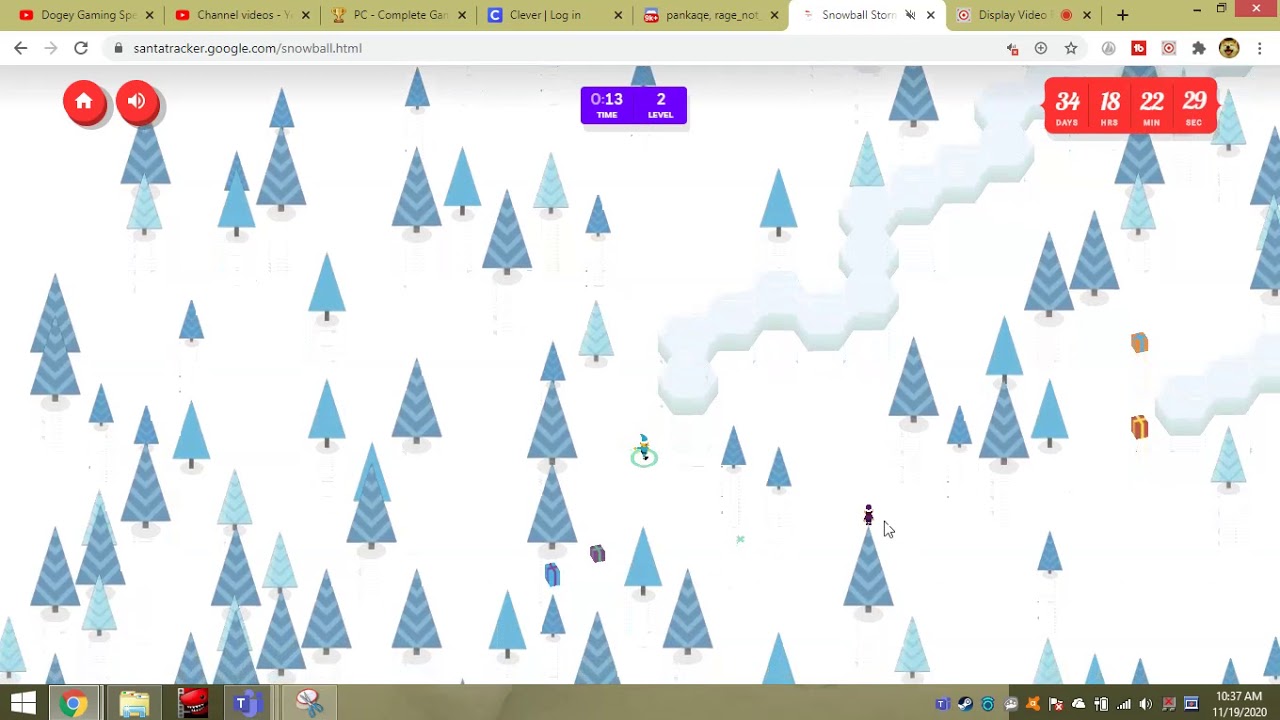This image is a detailed screenshot from the Doogie Gaming channel featuring a Santa Tracker interface. It shows a live tracking of Santa Claus, complete with days, hours, and minutes counting down until his arrival. The central portion of the screen displays an expansive digital forest of AI-generated pine trees, with various people walking through them. Scattered among the trees are numerous wrapped presents. In the background, a white slope—possibly a ski trail—adds depth to the scene as objects cascade down it. The bottom part of the interface seems to display video content, potentially from the game the user was playing or a related commentary, marked by references to Doogie Gaming channel videos, PC completion, and a clever login package. The ensemble of digital elements creates a festive yet dynamic portrayal of the holiday countdown.